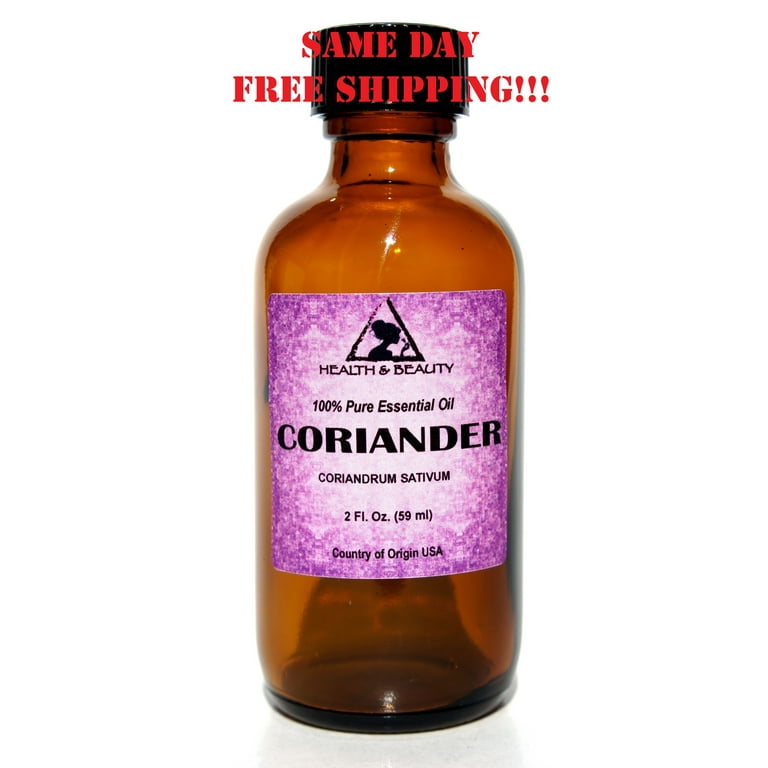This product photograph features an amber-colored glass bottle with a ridged black screw-top cap, filled with a clear liquid up to its neck. The bottle is designed to appear as if it is floating in a featureless white void, typical for online commercial listings. The bottle bears a lavender label that fades to white towards the center, with a triangular logo at the top featuring a silhouette of a woman applying makeup. Below the logo, the black printed text reads, "Health and Beauty, 100% pure essential oil, Coriander, Coriandrum sativum, 2 fluid ounces (59 milliliters), Country of origin: USA." Prominently displayed in red text at the top of the image are the words “same day free shipping!!!”